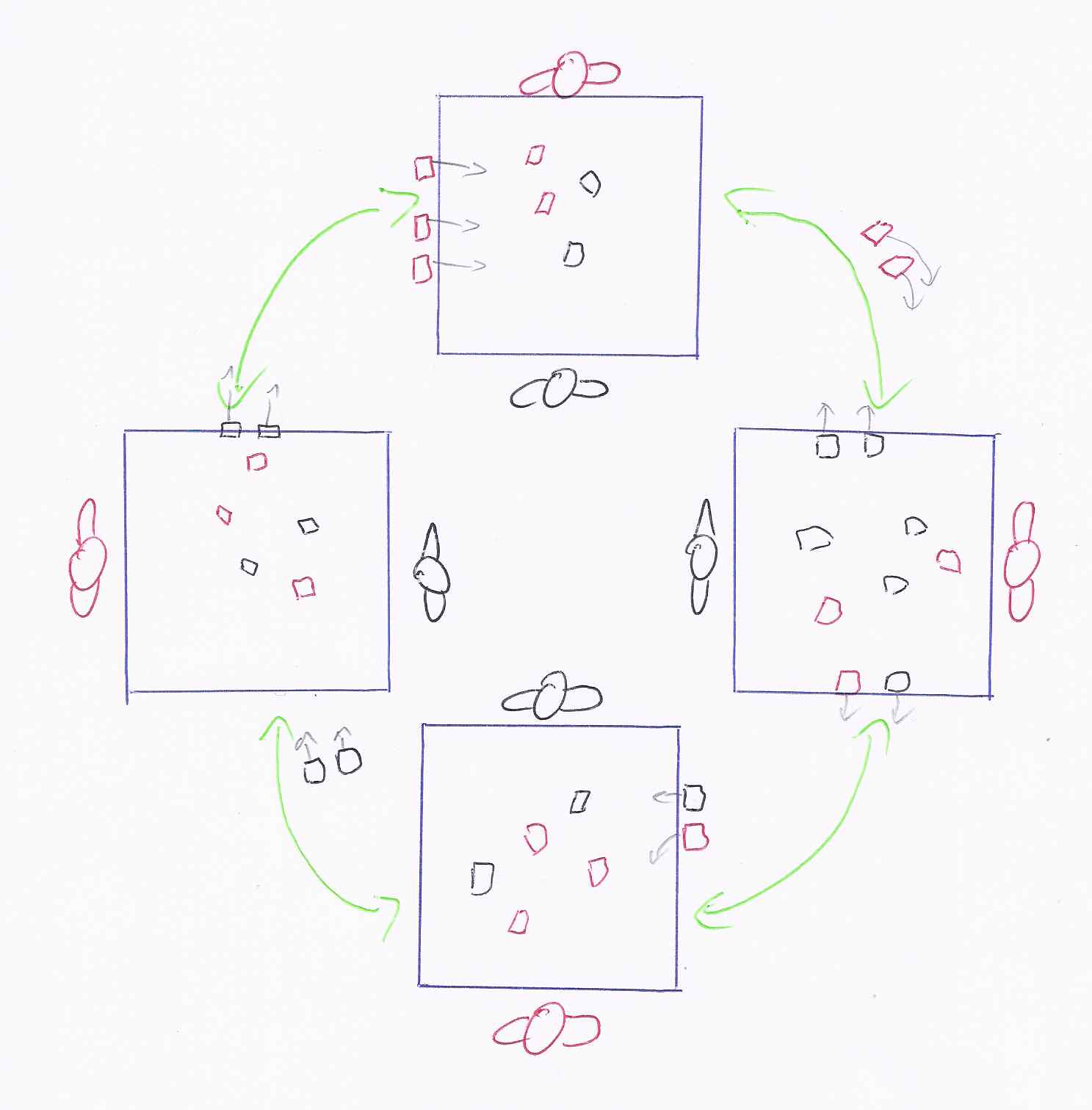This image portrays a detailed diagram consisting of four squares arranged in a 2x2 grid on a white background. Each square contains various geometric shapes that symbolize humans and possible markers or objects. The connections and interactions among the squares are illustrated with green arrows, suggesting a sequential process or flow from step 1 to step 4. 

The squares, outlined in blue, represent distinct areas or zones, possibly rooms or tables. Inside each square, red and black figures depict human-like shapes and other elementary geometric forms, though these figures are unlabeled and simplistic in design. 

The use of different colors aids in differentiating the elements: blue for the squares, green for the arrows indicating connections, and red and black for the human figures and other shapes. This color-coded visual plan effectively conveys the interaction and movement between the four distinct areas.